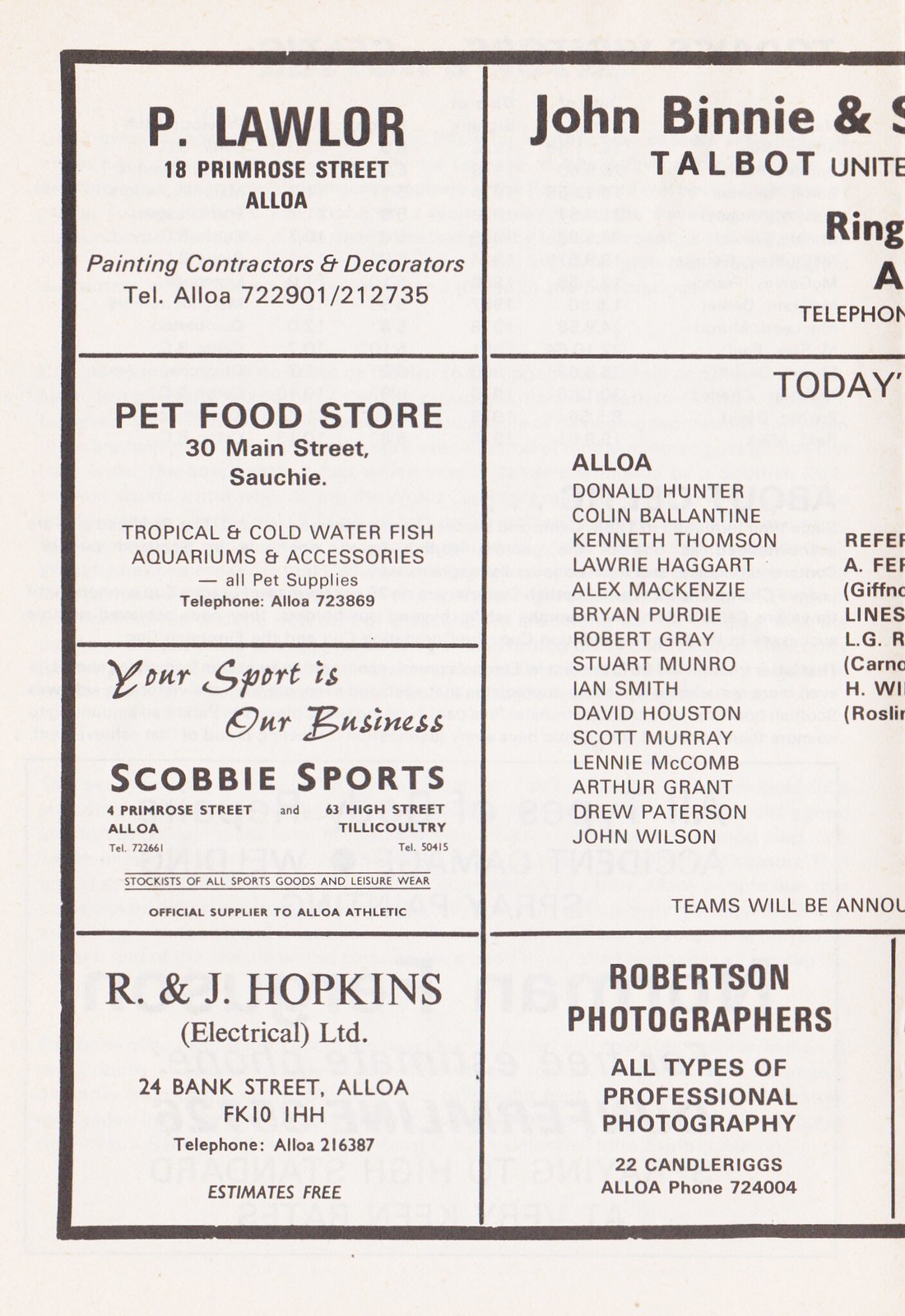This black-and-white image, resembling an old phone book or a printed program, displays a collection of advertisements mainly from various local businesses. On the left-hand side, there are four stacked squares: the top one for "P. Lawler" located at 18 Primrose Street, Aloa, advertising painting contractors and decorators with the telephone numbers Aloa 722901 and 212735; below it, a "Pet Food Store" at 30 Main Street, Sauchie, offering tropical and cold water fish, aquariums and accessories, and all pet supplies; followed by an ad for "Your Sport is Our Business, Scobie Sports," promoting sporting goods; and lastly, "R & J Hopkins Electrical Limited" at 24 Bank Street, Aloa, FK10 1HH, offering free estimates.

To the right of these ads, the image is partially cut off, revealing incomplete text that mentions "John Binney and" and "Talbot United." Below that, the text lists "today" and "LLOA," along with several names. In the bottom right corner, there's a large square for "Robertson Photographers," advertising all types of professional photography at 22 Candler Riggs, Aloa, with the phone number 724004. The overall grayish-tone image, bordered by clear separations between the ads, evokes a nostalgic feel suggestive of traditional print media.